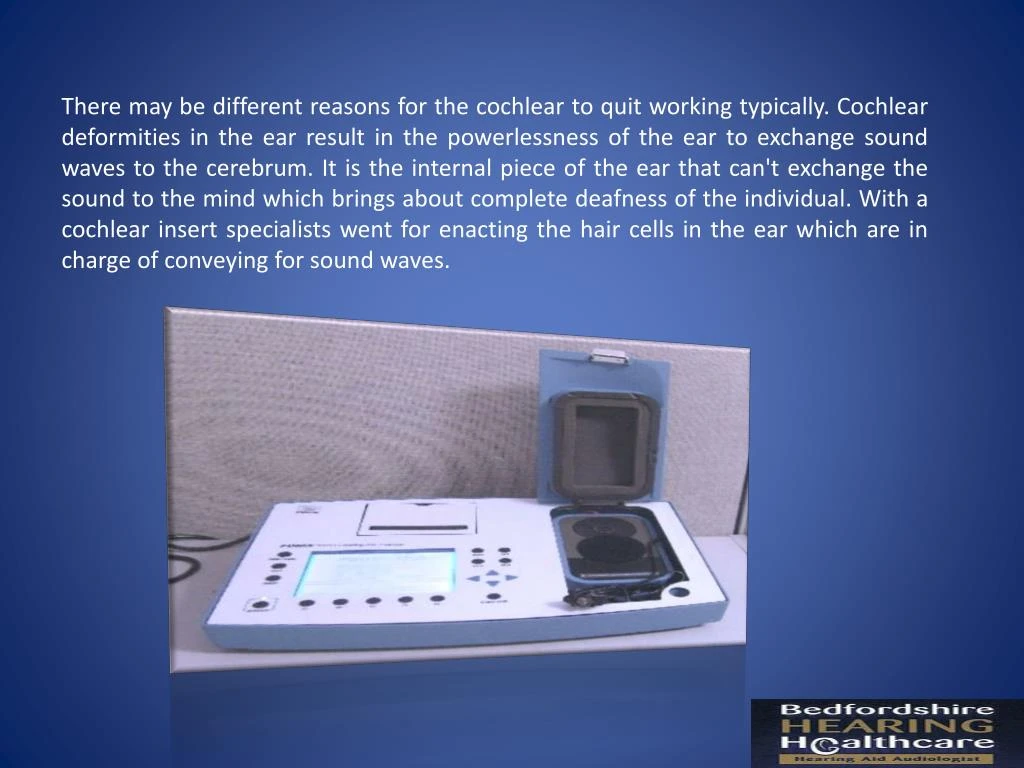The advertisement features a blue backdrop with a large block of white text at the top, detailing hearing impairments, specifically cochlear deformities that prevent sound waves from being transmitted to the brain, resulting in complete deafness. It mentions cochlear implants aimed at activating hair cells responsible for sound transmission. The central image showcases a sophisticated, flat, computerized medical device with numerous black buttons, arrow keys, and a large LCD screen on the left. On the right, there is an opened blue door featuring holes, a seal, gray foam chambers, and a clasp for secure closure. The device is positioned on a white table, backed by a gray board. The text appears to be a translation, possibly not originally in English, as the wording is somewhat unclear. The bottom right corner bears the logo "Bedford Shire Hearing Healthcare" alongside the name of the highlighted medical instrument.